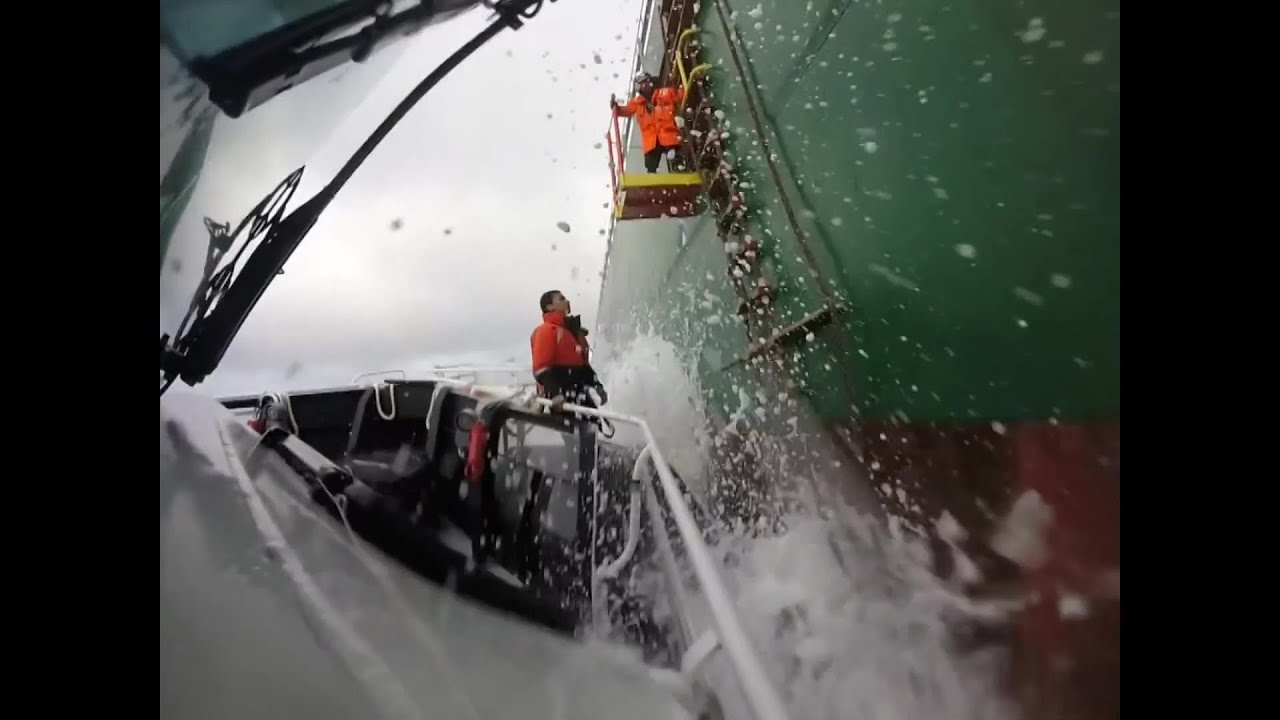The photograph captures a dramatic scene at sea amidst stormy weather, featuring two interconnected vessels. Central to the image is the green hull of a large ship, its lower section painted in a reddish maroon, creating a vivid contrast against the surging gray waters. A smaller white vessel, possibly a tender, approaches the larger ship, with water violently splashing between them.

The sky is overcast with dense, gray clouds indicating a storm, and the rough seas further contribute to the tumultuous atmosphere. On the large ship’s hull, a person clad in a fluorescent orange jacket and helmet is positioned midway on an external ladder attached to a yellow platform. His stance on the ladder suggests he is either ascending or descending as he tends to the task at hand.

On the smaller white vessel, another man, also wearing a bright orange jacket but without headgear, stands on the exterior side of the railing. He gazes up intently at his counterpart on the larger ship, his black mask resting around his neck. The proximity of the two vessels and the interaction between the men amidst the hostile environment contribute to the image’s stirring energy and narrative of cooperation in challenging conditions.